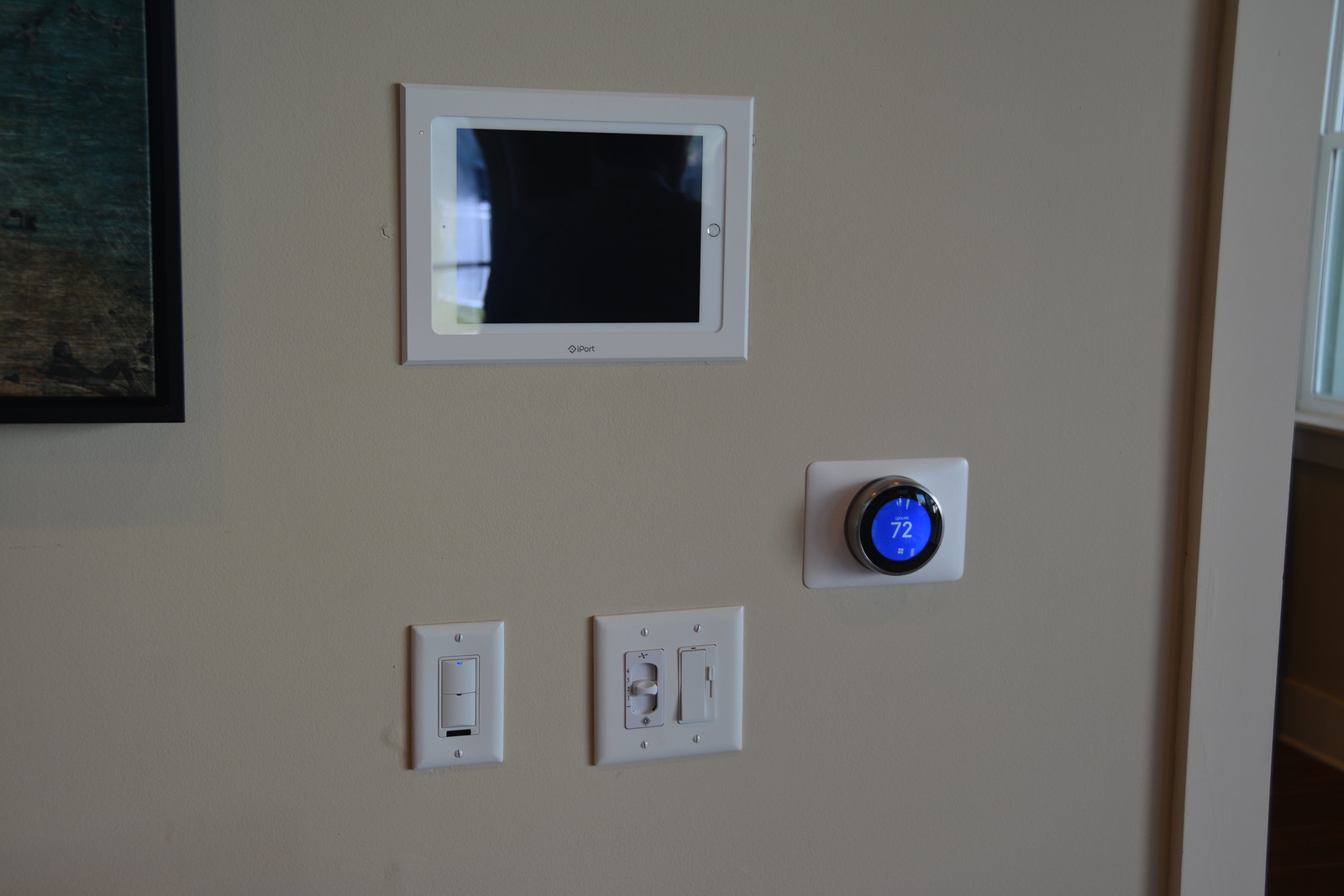This detailed color photograph showcases a section of a white wall adorned with various items. In the top left corner, a small portion of a picture in a dark black frame is visible, hinting at a dark-colored artwork or photograph that remains mostly obscured from view. 

Centrally situated on the wall is a horizontally placed iPad encased in a shiny white frame, labeled "iPort" at the bottom. Below the iPad, a white light switch with two buttons is present; the top button features a blue indicator light.

Further down and to the right, another unique light switch with a movable lever stands out, deviating from the typical design. Adjacent to this, a conventional lever-type light switch within a white casing secured by four screws is shown, with its lever pressed in at the top.

Towards the rightmost part of the image, a white square features a central round object, encased in silver with a blue screen. This appears to be a smart home thermostat displaying "72" in the center of its screen, likely indicating the current temperature setting.

Each element on this wall contributes to the overall advanced and modern aesthetic captured in this photograph.